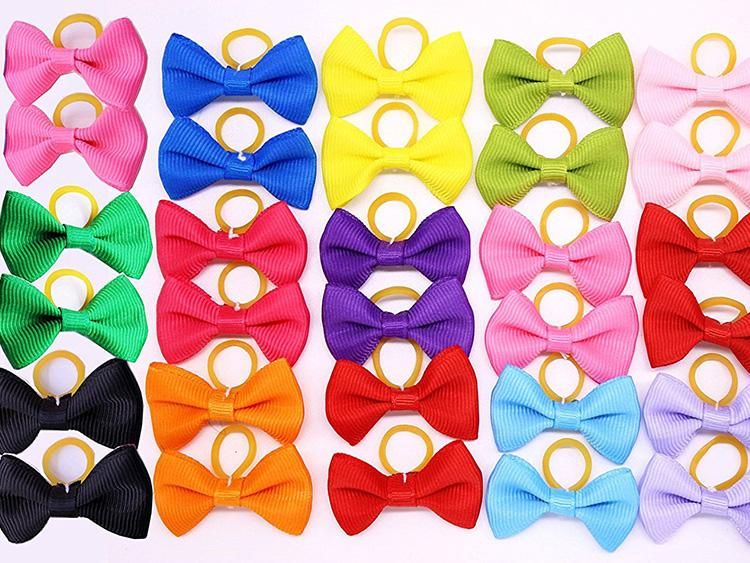The image features a neatly organized display of ribbon hair ties arranged in a structured grid pattern against a white background, which might be either a wall or countertop. Each set consists of two identical hair ties, with five columns and six rows completing the arrangement. The colors of the ribbons are laid out as follows from top to bottom starting from the first column: pink, green, black; the second column: blue, red, orange; the third column: yellow, purple, red; the fourth column: lime green, pink, light blue; and the final column: soft pink, red, lavender. Each hair tie is looped through a small rubber circle at the top, creating a visually appealing and colorfully diverse collection of bow-inspired hair accessories.